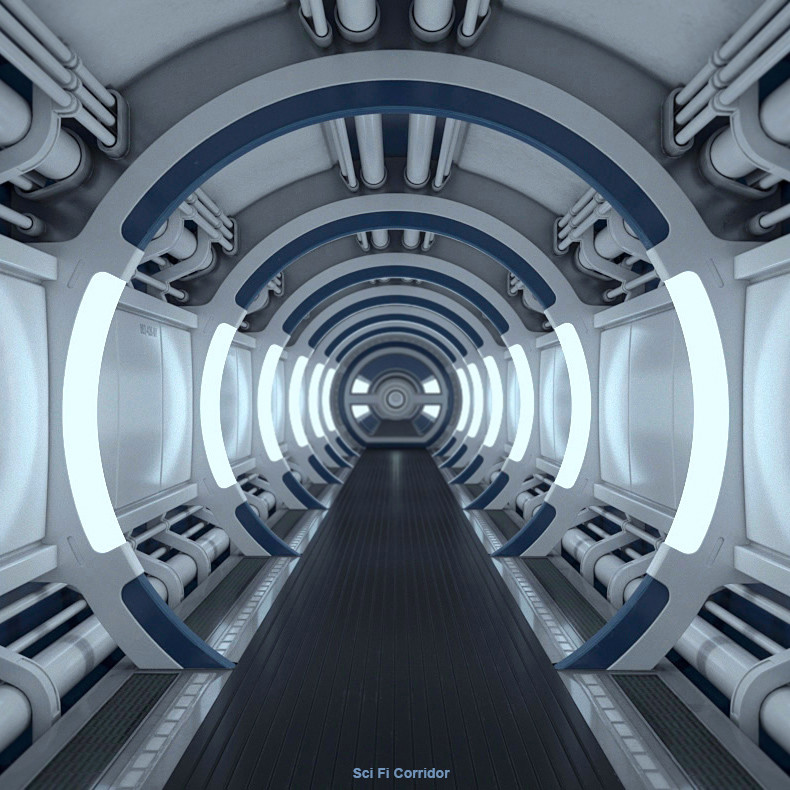This is a highly detailed, computer-generated illustration depicting the interior of a futuristic spaceship, reminiscent of the iconic spacecraft seen in Star Wars. The scene centers on a long corridor, featuring a sleek, black, plastic-like floor. The corridor's hallways are rounded, framed by a series of circular arches that extend into the distance. 

Lining these arches are brilliant white lights, casting an ethereal glow along the corridor's length. At the far end of the corridor stands a closed, circular hatch or door, signifying the pathway's conclusion. The ceiling and floor are intricately detailed with gray-colored steel pipes, adding to the industrial, high-tech ambiance. The walls flanking the corridor are crisp white, further illuminated by the central circular lights that spiral down the passage.

Amidst the detailed structure, the small text at the bottom of the image reads "sci-fi corridor," grounding the viewer in the genre of the scene.